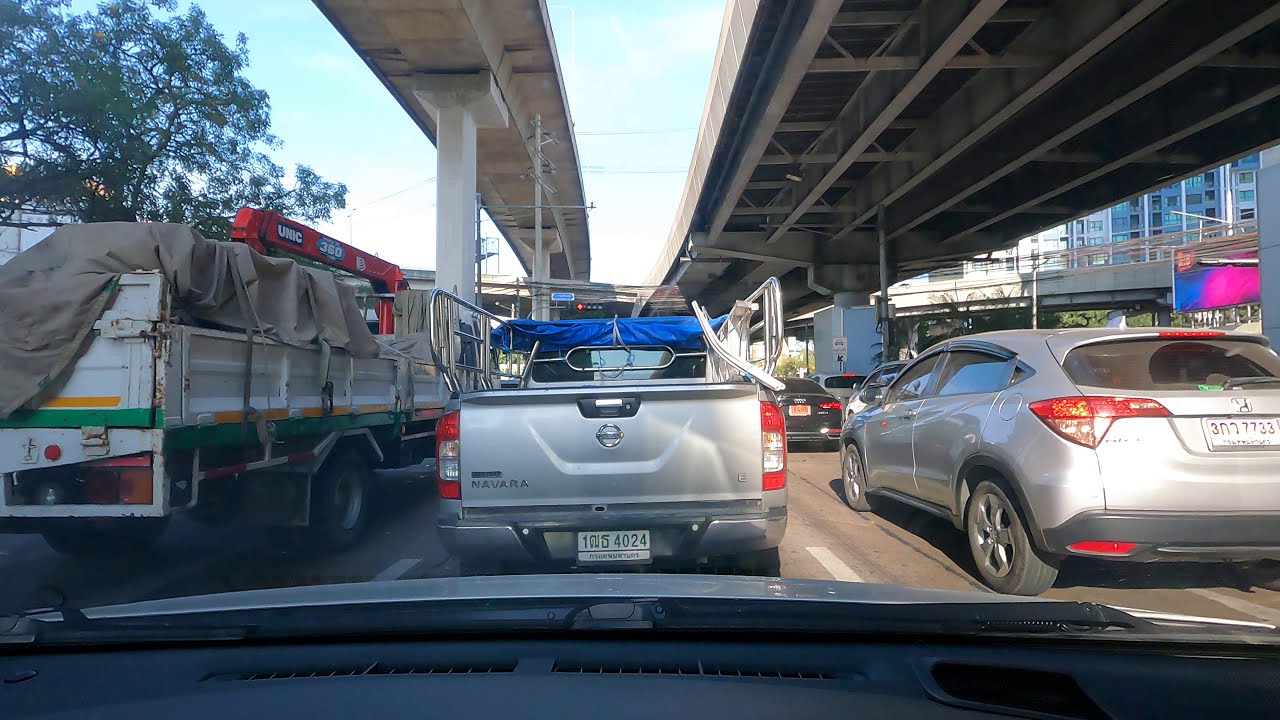The image captures a bustling city scene, with traffic visible from inside a car. The perspective from the dashboard and windshield reveals a road with at least three lanes filled with vehicles waiting at a traffic light. In the left lane, there's a large utility work truck, while the middle lane features a silver pickup truck, and the right lane has a silver SUV. Above the roadway, there's an elevated highway, suggesting heavy traffic both at ground level and above. To the right of the image, a skyrise building and a billboard are visible, while trees line the left side. The scene is set during the daytime amidst a typical city traffic jam.